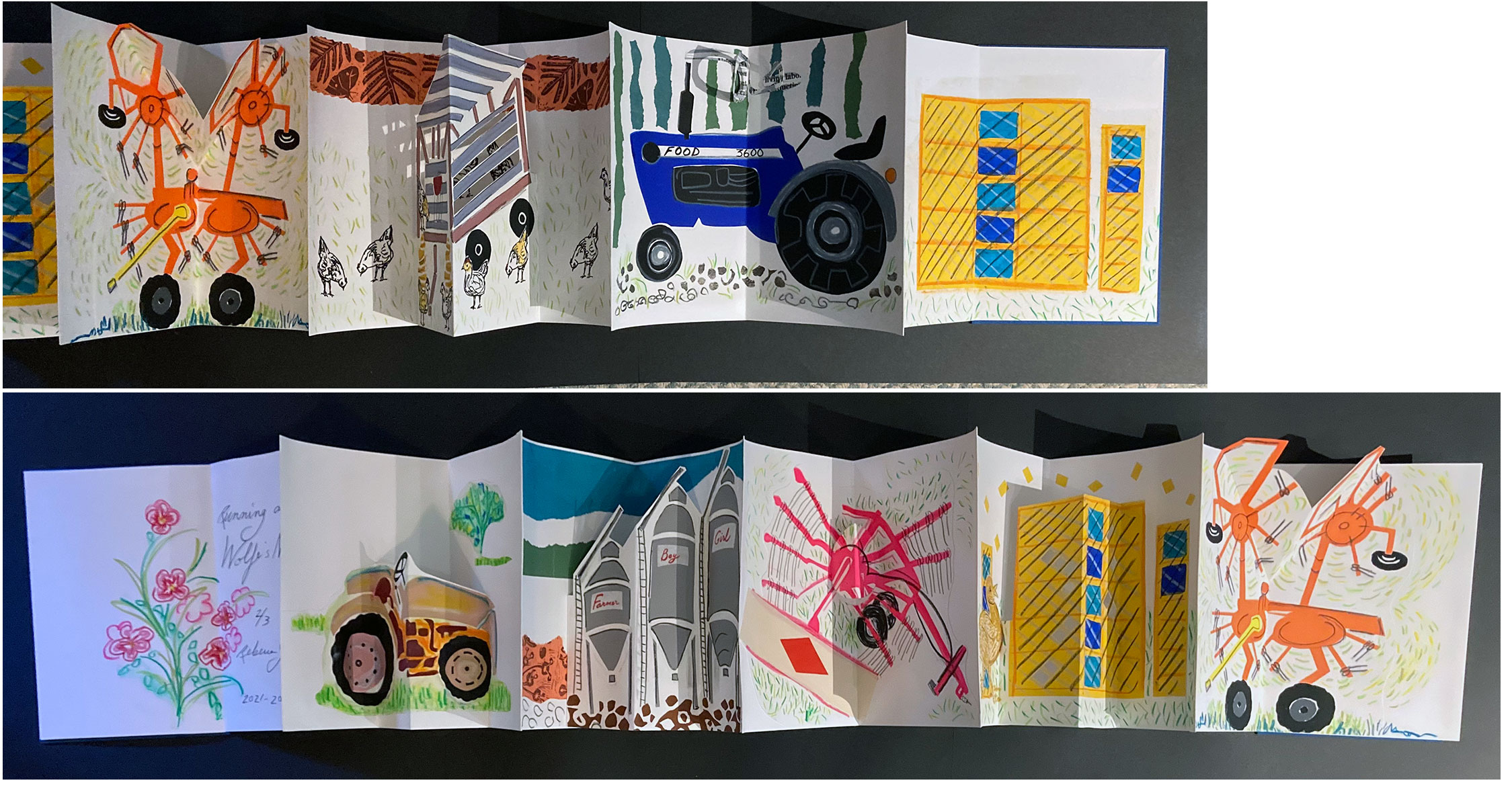The image showcases a homemade greeting card, uniquely crafted with various illustrations arranged in two columns, likely created by middle school children. The card features a series of paintings with a common farm theme. On the top row, from left to right, the first painting depicts an abstract object with wheels and a lever, resembling a deconstructed construction machine. The second illustration shows chickens in a farm setting, surrounded by grass and leaves. Next, there's a painting labeled "food 3600," featuring a large tractor amidst green grass. The fourth image appears to be a farm building, while the fifth remains partially obscured and indiscernible. The bottom row mirrors the top with slight variations; it starts with a painting of flowers, followed by a different tractor, a new factory illustration, and a pink object. Despite the repetition of the building and the deconstructed tractor, each section of this card is distinct, vibrant, and thoughtfully composed, making it a one-of-a-kind birthday or celebratory greeting card.